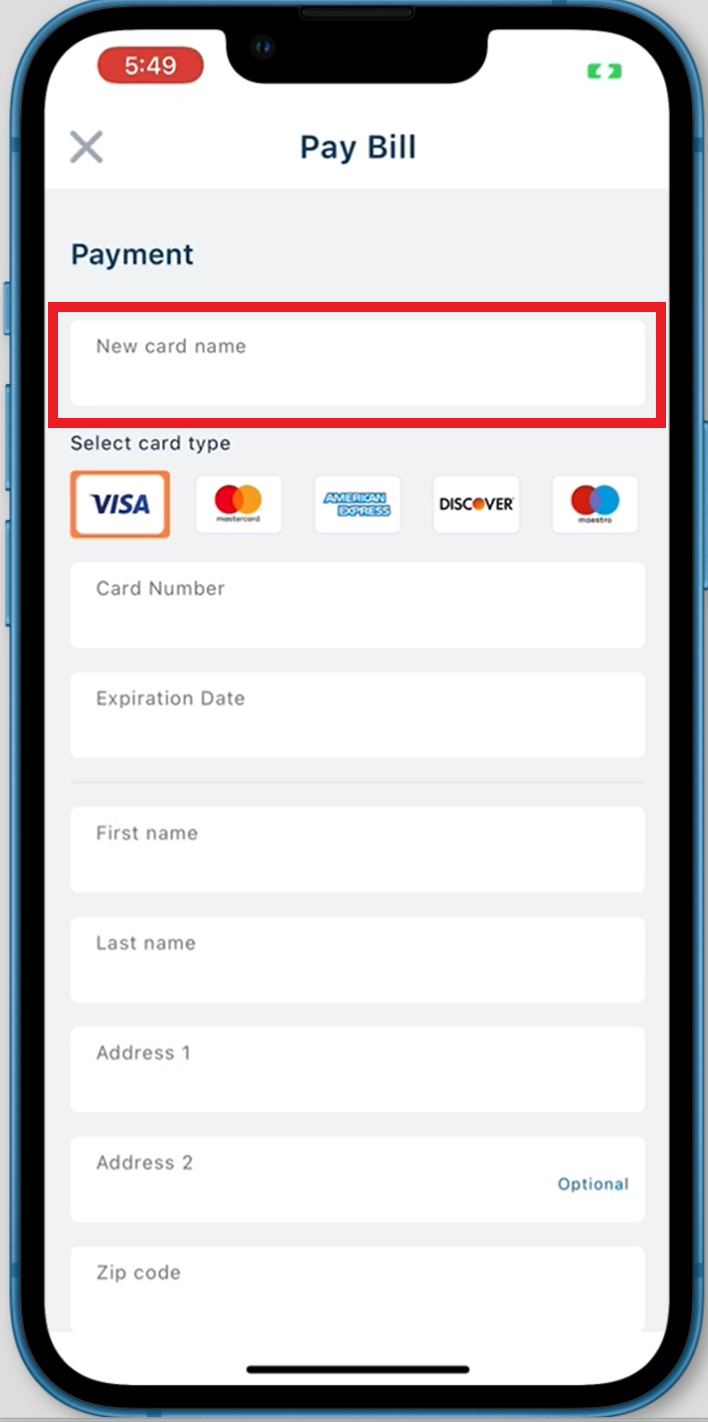This image depicts a blue smartphone, fully visible, featuring various elements on its screen. The device has buttons on the left side, including the sound, power, and sleep buttons. At the top of the phone, there's a camera. 

On the screen, the time is displayed at the top left, reading 5:49, outlined in a red oval with white numerals. The top right shows a battery icon. Directly under the top icons, there is the text "Pay Bill" with an "X" to the left of it. Below that, it reads "Payment" followed by a text box labeled "New Card Name," which is outlined in a red box.

Further down, the phone screen shows a dropdown menu with the label "Select Card Type." The options listed include Visa, MasterCard, American Express, Discover, and Maestro, with Visa selected and outlined in an orange box. 

Below this dropdown are several text boxes labeled respectively as "Card Number," "Expiration Date," "First Name," "Last Name," "Address," "Address 2" (the latter of which is marked as "optional" in blue text on the right), and "Zip Code."

At the very bottom of the screen, a black line suggests a possible upward swipe action to access a hidden menu. The phone appears to be resting on a white surface, which is visible in the corners of the image.